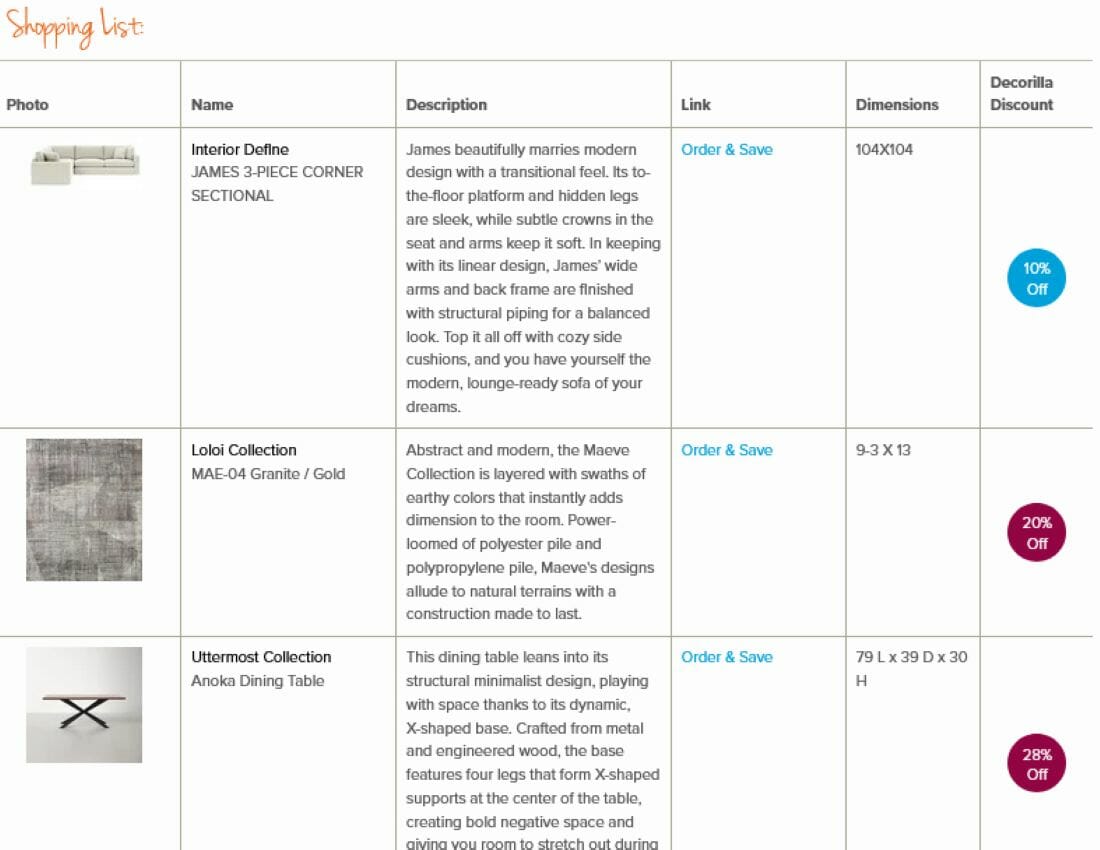In the top left corner of the chart, there is a heading in orange text that reads "Shopping List". The chart itself consists of multiple columns labeled from left to right as follows: "Photo," "Name," "Description," "Link," "Dimensions," and "Decorilla Discount."

The first row, under "Photo," features an image of a white sectional couch. Adjacent to it, under "Name," is the text "Interior Define James Three-Piece Corner Sectional." In the "Description" column, there's a detailed paragraph describing the item. The "Link" column includes the text "Order and Save" in blue, signifying a clickable option. For dimensions, it states "104 x 104," and under the "Decorilla Discount" column, there's a blue circle with "10% off" written in it.

In the second row, the "Photo" column depicts a texture that is not clearly identifiable. The "Name" column reads "Loy Collection May 04 Granite Gold." A detailed description follows in the next column. The discount here is noted as "20% off."

The final row shows an image of a dining table under the "Photo" column. The "Name" column labels it as "Uttermost Collection Good Dining Table." Following a description, the "Link" column again features the text "Order and Save" in blue. The dimensions for this table are listed as "79 L x 39 D x 30 H." The "Decorilla Discount" column indicates a discount of "28% off."